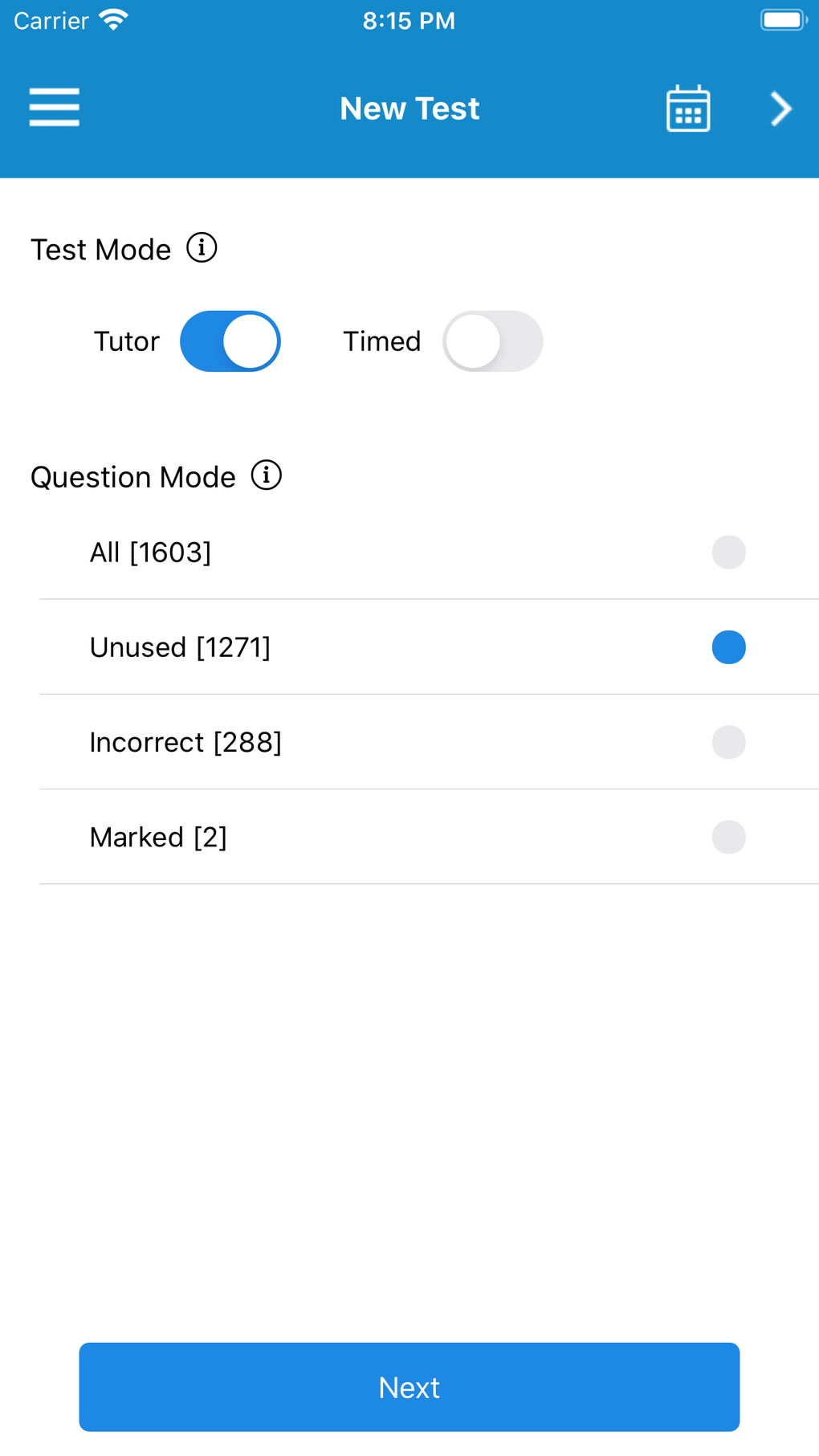This portrait-format, color screenshot captures the display of a mobile phone. The status bar at the top reveals various details: the mobile phone provider is Carrier, the time is 8:15 PM, and the battery is fully charged. A prominent blue banner at the top displays the text "New Test" in white lettering. To the right of this banner, a calendar icon is visible, suggesting an option to schedule or view dates.

The main section of the screen emphasizes a "Test Mode" feature, accompanied by an information icon (a small "i") that offers additional details when tapped. Two primary modes are available for selection: "Tutor" and "Timed," with the "Tutor" mode being currently activated.

Below this, a heading labeled "Question Modes" presents four options with corresponding question counts:
- "All" with 1,603 questions
- "Unused" with 1,271 questions, which is currently selected
- "Incorrect" with 288 questions
- "Marked" with 2 questions

Considering the selections made ("Unused" ticked under Question Modes and "Tutor" mode activated), the interface now provides a "Next" button at the bottom, ready to proceed to the next step.